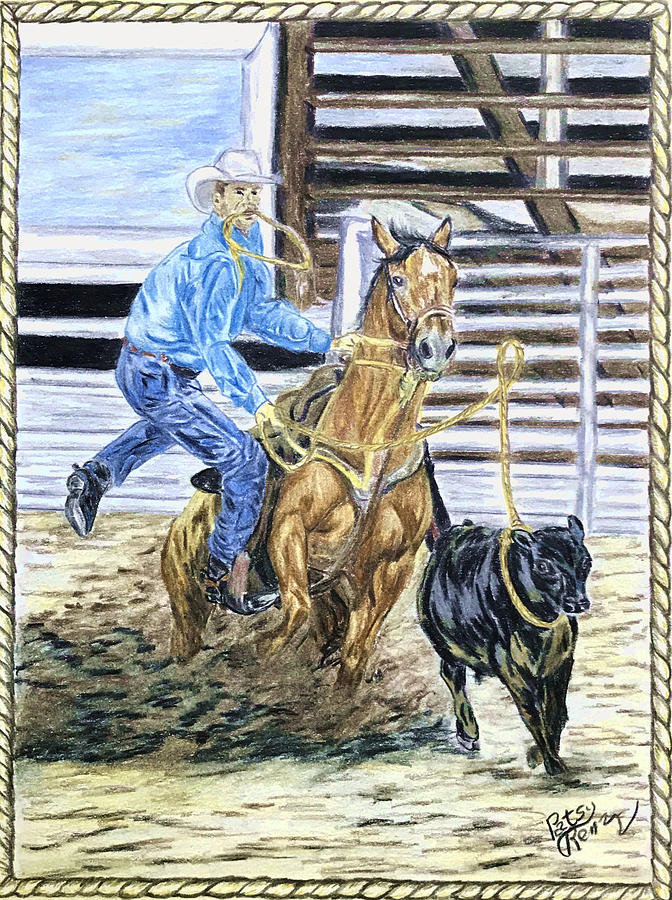This is a detailed drawing, possibly created with pastels, colored pencils, or even crayon. The artwork depicts an action-packed rodeo scene. Central to the image is a cowboy, wearing a white cowboy hat, a denim-colored shirt, blue jeans, and black cowboy boots. The cowboy, who is Caucasian with fairly pale skin, is in the midst of lassoing a young calf. He holds a brown rope in his hand and also bites down on part of the rope. The light brown horse, marked with a small white patch on its forehead, gallops vigorously, kicking up a storm of brown dust. The black calf, with some brown patches on its legs, has been successfully roped and runs ahead of the horse. Surrounding this dynamic scene is a hand-drawn border resembling a rope, giving the artwork a framed appearance. The artist's signature is placed in the lower right-hand corner, though it is too small to discern.